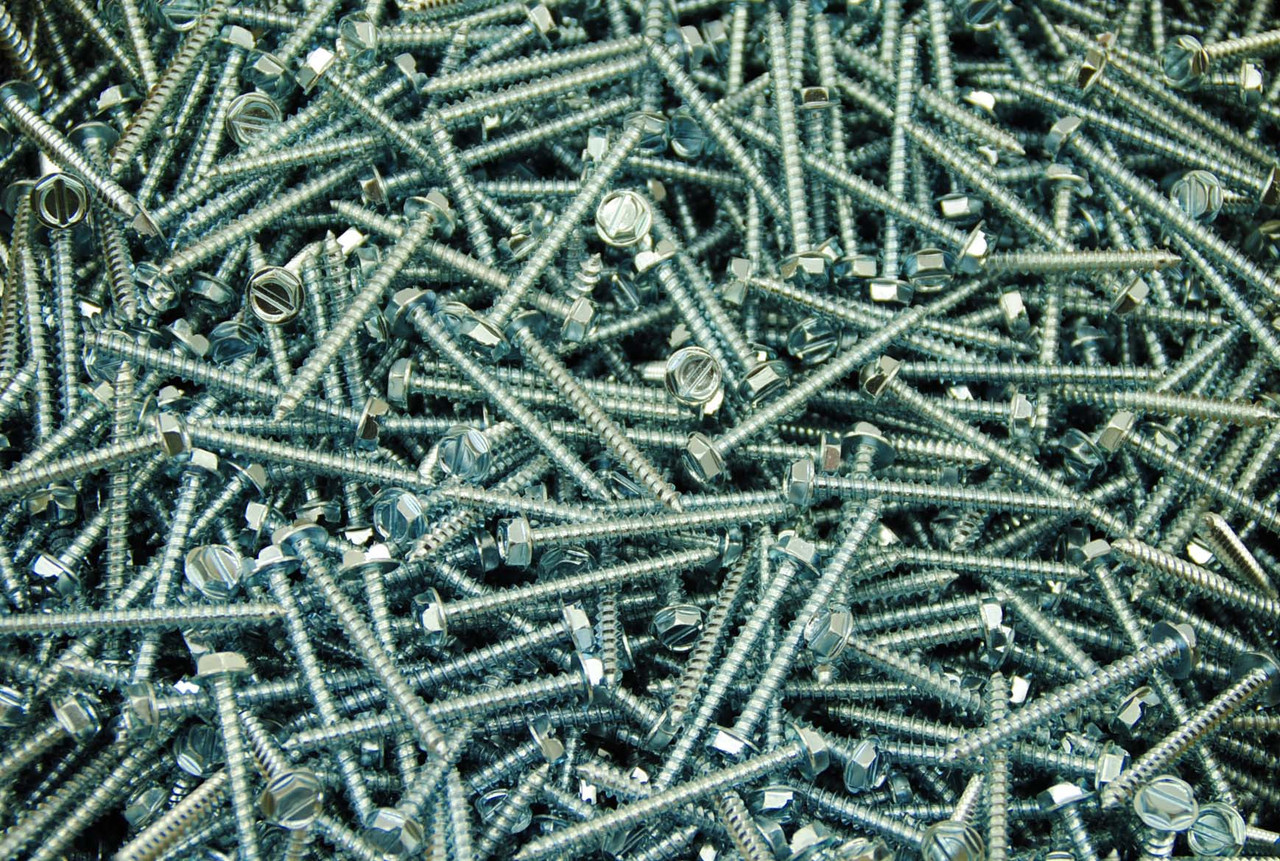The image shows a detailed, close-up view of a large, deep pile of screws, all of which appear to be new and uniformly silver in color. The screws are approximately 3 inches in length and feature a straight edge across the top, indicating they would require a flathead screwdriver for use. Most of the screws are laid on their side, with some pointing in various directions—up, down, left, and right. A few screws are positioned upright, allowing a clear view of their hex heads, but the majority are partially obscured within the heap. The pile appears to be very deep, with no visible surface or table beneath it.